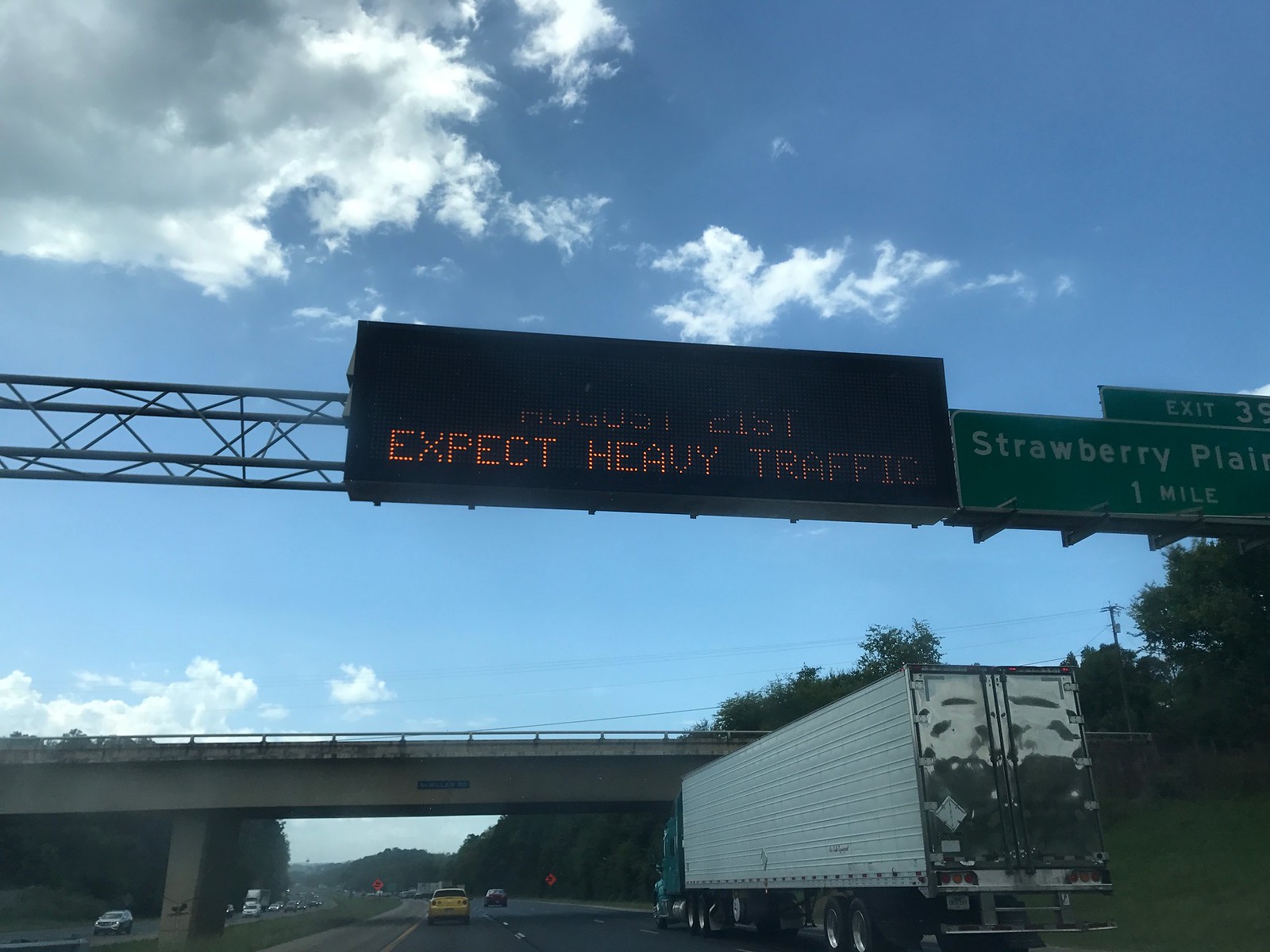The image captures a freeway scene from a driver's perspective, prominently featuring a black digital sign mounted on horizontal poles. The sign displays the message "August 21st, expect heavy traffic" in bright digital text. To the right of this sign is a partially visible green sign that reads "Exit 30, Strawberry Plain, one mile." The highway stretches off into the distance, curving slightly to the left, and is framed by a concrete overpass. Vehicles populate the road, including a large semi-truck with a green cab and white storage area on the right, a yellow car ahead, and a red car in the adjacent lane. In the distance, more cars and trucks are visible on both sides of the overpass. The sky above is a clear blue with a few scattered clouds, suggesting a sunny day. The scene is bustling with traffic and rich in detail, capturing the essence of a busy freeway.